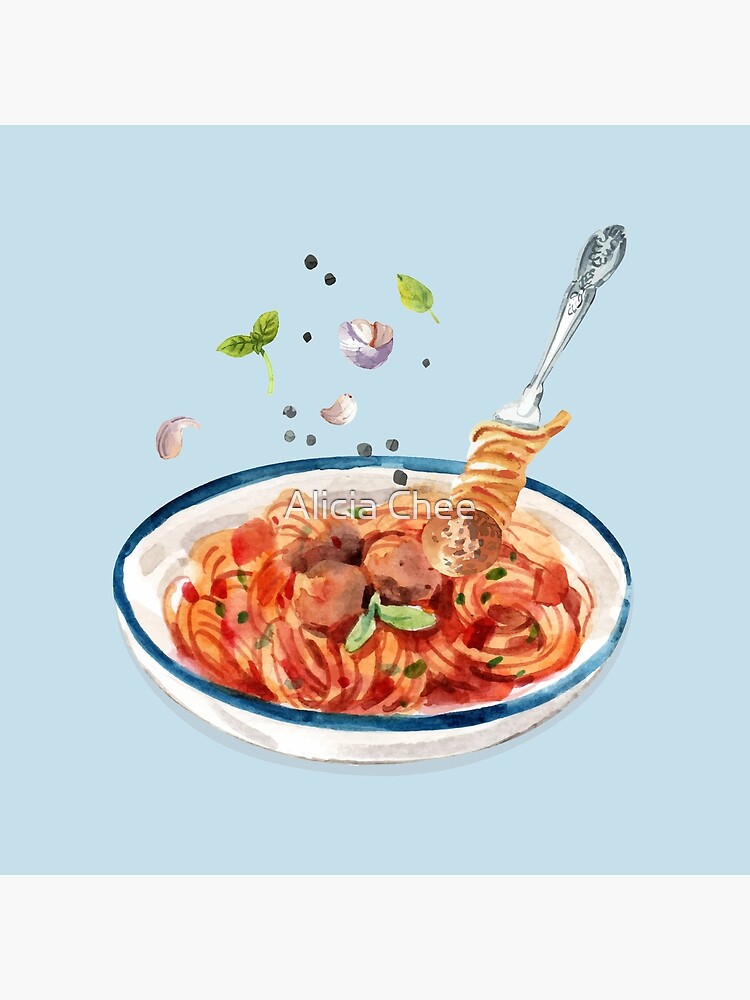A beautifully detailed watercolor illustration depicts a plate of spaghetti and meatballs set inside a white bowl with a blue rim. The twirled pasta is generously coated with tomato sauce, and you can see chunks of tomato interspersed among the strands. In the center of the dish, three delicious meatballs are nestled, surrounded by hints of onions and green leaves, possibly basil or oregano. Hovering above the bowl are additional garlic cloves, basil leaves, and a scattering of pepper flakes, as if freshly sprinkled. A fork, poised to take a bite, has twirled some pasta and speared one of the meatballs. The composition is gracefully set against a light blue background, capturing the essence of a homely, yet elegant meal. The artwork is signed with a watermark reading "Alicia Chee, C-H-E-E" in the middle of the image.